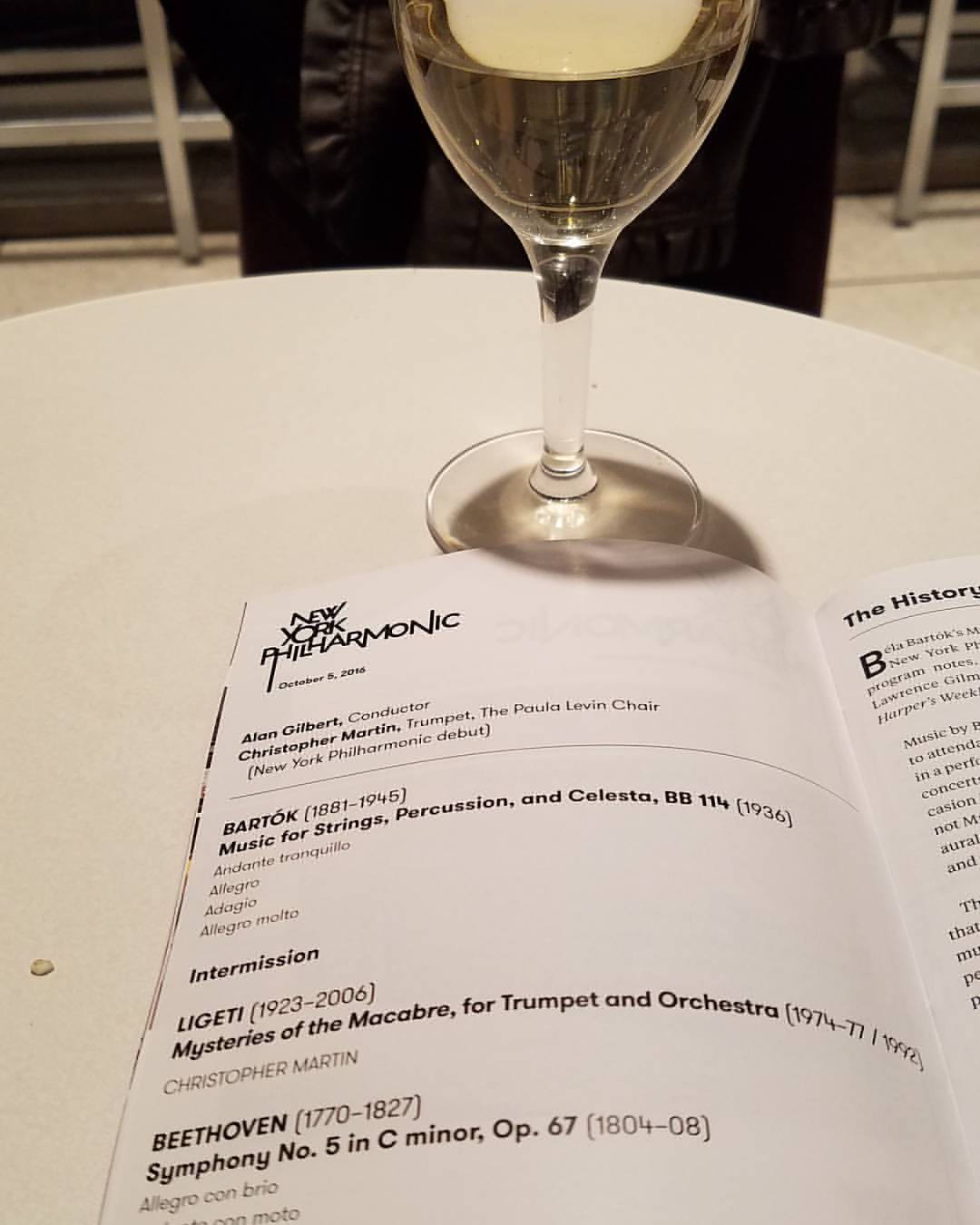In a well-lit restaurant or winery setting, a color photograph in portrait orientation captures a detailed scene showcasing a white round table. Centrally positioned on the table is an open, black-and-white musical program from the New York Philharmonic with a distinctive modern, all-caps font on the top left, dated October 5, 2016. The program credits Alan Gilbert as the conductor and Christopher Martin on trumpet, noting his New York Philharmonic debut. Listed musical selections include works by Bartók, Ligeti, and Beethoven, with an intermission interspersing the performance. In front of this handbill sits a half-full stemmed wine glass containing white wine. The background reveals a distant chair draped with a coat, hinting it may be a concert area possibly in a balcony section, indicated by a visible barrier that resembles a gate. The carpeted floor area complements the intimate, refined ambiance projected by the overall image.